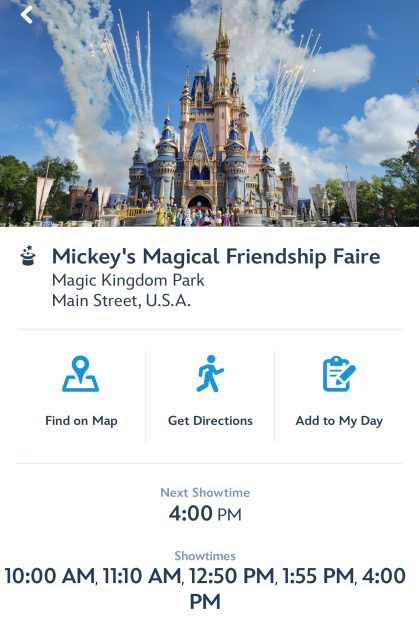In this vibrant photograph captured at Magic Kingdom Park, part of Walt Disney World Resort in Florida, we see the enchanting scene of "Mickey's Magical Friendship Fair" taking place on Main Street, USA. The iconic Cinderella Castle stands majestically at the center, framed by lush green trees on either side. The sky is a brilliant blue, dotted with delicate white clouds, which adds to the enchanting atmosphere of the fair.

Above the castle, colorful fireworks burst into brilliant displays, leaving trails of smoke behind and illuminating the sky with festive lights, capturing the very essence of Disney magic. The image portrays a cheerful and inviting ambiance, enticing visitors to experience the show.

Text overlays inform guests about the various showtimes for "Mickey's Magical Friendship Fair," specifically noting performances at 10:00 AM, 11:10 AM, 12:50 PM, 1:55 PM, and the final show at 4:00 PM. Interactive options are also visible, allowing potential attendees to find the show on a map, get directions, or add the event to their day's itinerary.

This photo brilliantly encapsulates the allure of Disney's live performances, urging viewers to immerse themselves in the delightful spectacle that awaits at the heart of Magic Kingdom Park.